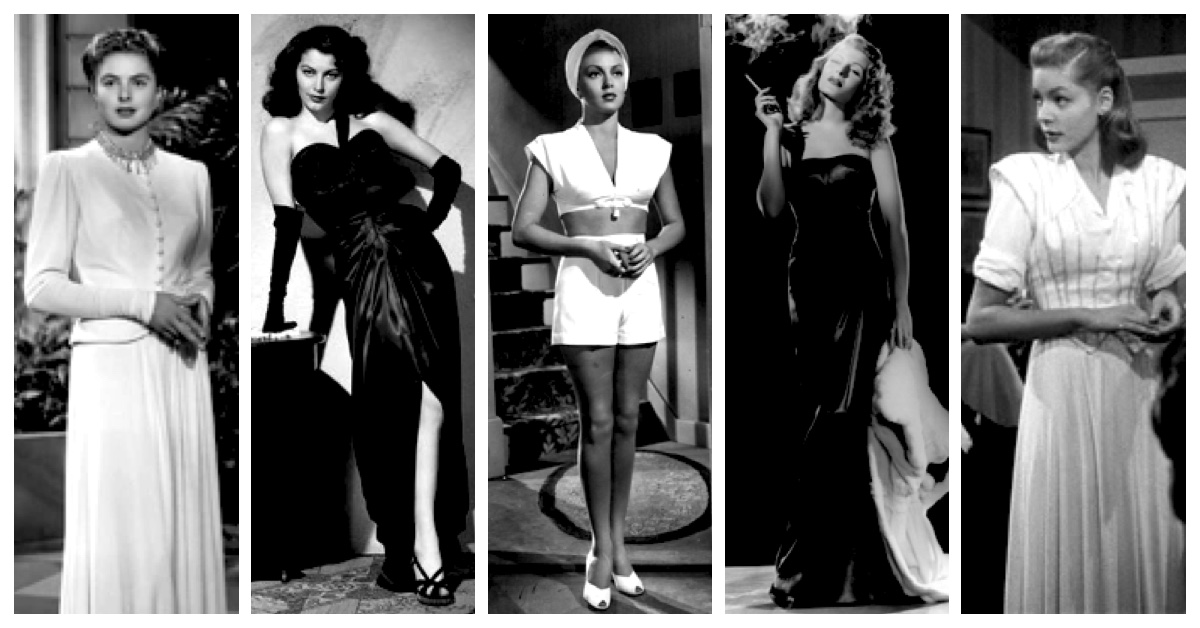The image is a series of five black-and-white photographs, each capturing a different woman in a distinct scene, split into five sections from left to right. These women emanate a vintage, classy aura reminiscent of the 1930s to 1950s.

Starting on the far left, the first woman is dressed in a long-sleeve white dress, her short or neatly pulled-back hair accentuating her reserved elegance as she looks slightly to the side, her hands clasped gently in front of her.

The second woman exudes glamour with her long black hair and slight smirk aimed directly at the camera. She is draped in a strapless black evening gown that features a slit, revealing her leg. Her ensemble is completed with high heels and elbow-length black gloves, emphasizing her sophisticated, high-society look. 

In the center, the third woman is portrayed in a white ensemble comprising a crop top, short shorts, and high heels, topped off with a white headpiece. Her exposed legs and poised stance, hands clasped in front of her, indicate a chic, daring fashion sense of the time. She is positioned in front of a staircase, adding depth to the scene.

The fourth woman, radiating sultry allure, tilts her head back slightly as she smokes a cigarette, the smoke lingering above her. She wears a strapless black evening gown and has dimly lit, potentially blond hair. In her left hand, she holds a white fur stole, contributing to her glamorous and slightly provocative appearance.

The fifth and final woman on the far right presents a more modest demeanor. She is clad in a long, formal white dress with long sleeves. Her gaze is directed to the left, and her hands are delicately clasped in front of her, embodying refined grace.

All five women, portrayed in these monochromatic images, beautifully encapsulate the vintage sophistication and diverse fashion of their era.